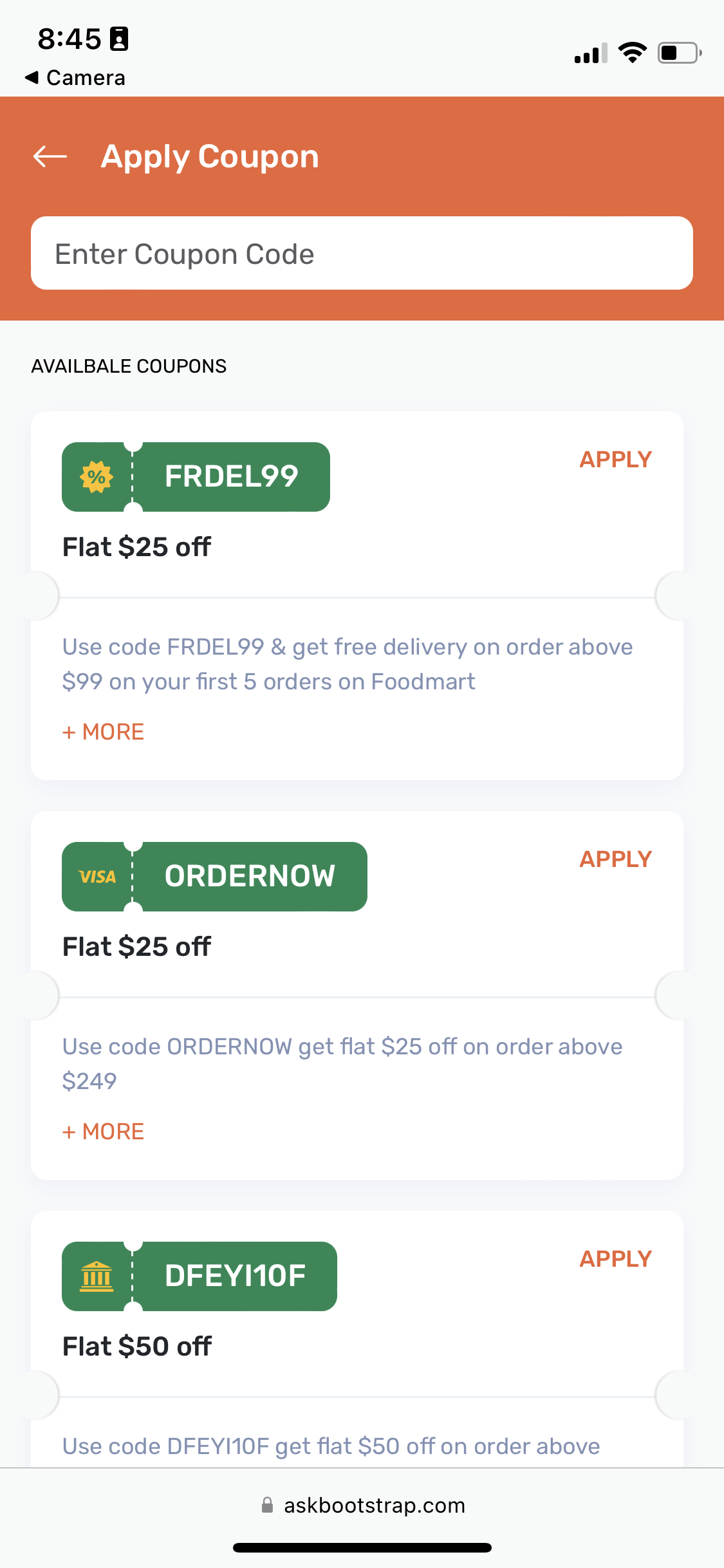A user navigates a coupon application section on the website askbootstrap.com. They are presented with various discount offers for Food Mart. The first coupon offers a flat $25 discount on orders over $99, applicable for the first five orders. The second coupon provides a $25 discount on orders exceeding $249. The third coupon mentions a $50 discount although the specifics of the minimum order requirement are not fully visible. All coupon codes are highlighted in green, and each has an orange 'Apply' button next to it. The image appears to be taken on a mobile device with low battery but strong Wi-Fi signal, and the timestamp reads 8:45, which could be either AM or PM. The layout and functionality of the website resemble those of the Honey discount extension.